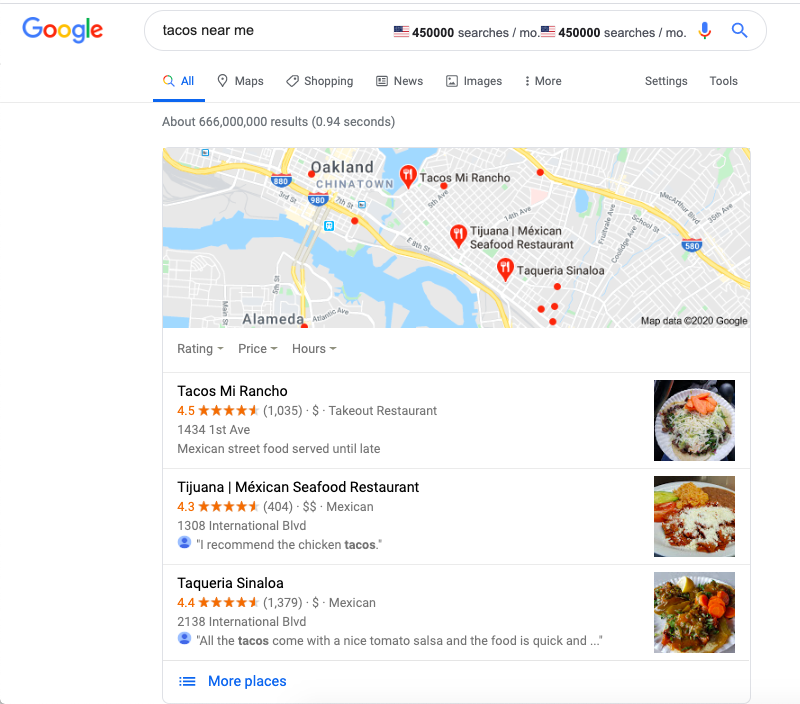The image depicts a Google search results page with the query “tacos near me,” prominently displayed at the top within a white search bar. The Google logo is featured on the left side of the bar, with each letter in its distinctive colors: a blue ‘G’, red ‘o’, yellow ‘o’, blue ‘g’, green ‘l’, and red ‘e’. Below the search bar, it’s noted that there are approximately 450,000 searches per month for this query.

Directly below, in blue and underlined, is the word "All," indicating the current tab. Other tabs such as "Maps," "Shopping," "News," "Images," and "More" are listed in black. Further right, "Settings" and "Tools" are also present, separated by a thin gray line across the page.

The next segment of the image is a map, which details various notable locations and routes. Blue denotes water bodies, orange represents highways, and the land areas appear in shades of orange and gray. Streets are depicted in white with black text labels. Several locations are identified, including Oakland, Chinatown, Coolidge Avenue, School Street, and MacArthur Boulevard.

Beneath the map, search results list three local restaurants known for their tacos. The first is "Tacos Mi Rancho," followed by "Tijuana Mexican Seafood Restaurant," and finally "Taqueria Sinaloa." Additional details about rates and operating hours are also mentioned.